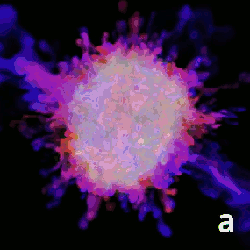The animated image features an ever-changing celestial scene set against a black background. It alternates between two states labeled by letters at the bottom right: A and B. The image under label A portrays a vibrant starburst or sunburst, depicted in shades of bright and dark pink with spiky lines radiating outward, suggesting an explosive energy. In contrast, B represents a more condensed and globular form, a nucleus-like ball of energy, blending darker hues of blue, purple, and black with touches of white and yellow. The colors range widely across the spectrum, including reds, greens, and pastels, giving the animation a dynamic and shifting appearance that resembles scientific visualizations of stellar phenomena, possibly depicting stages of a star or sun going supernova.